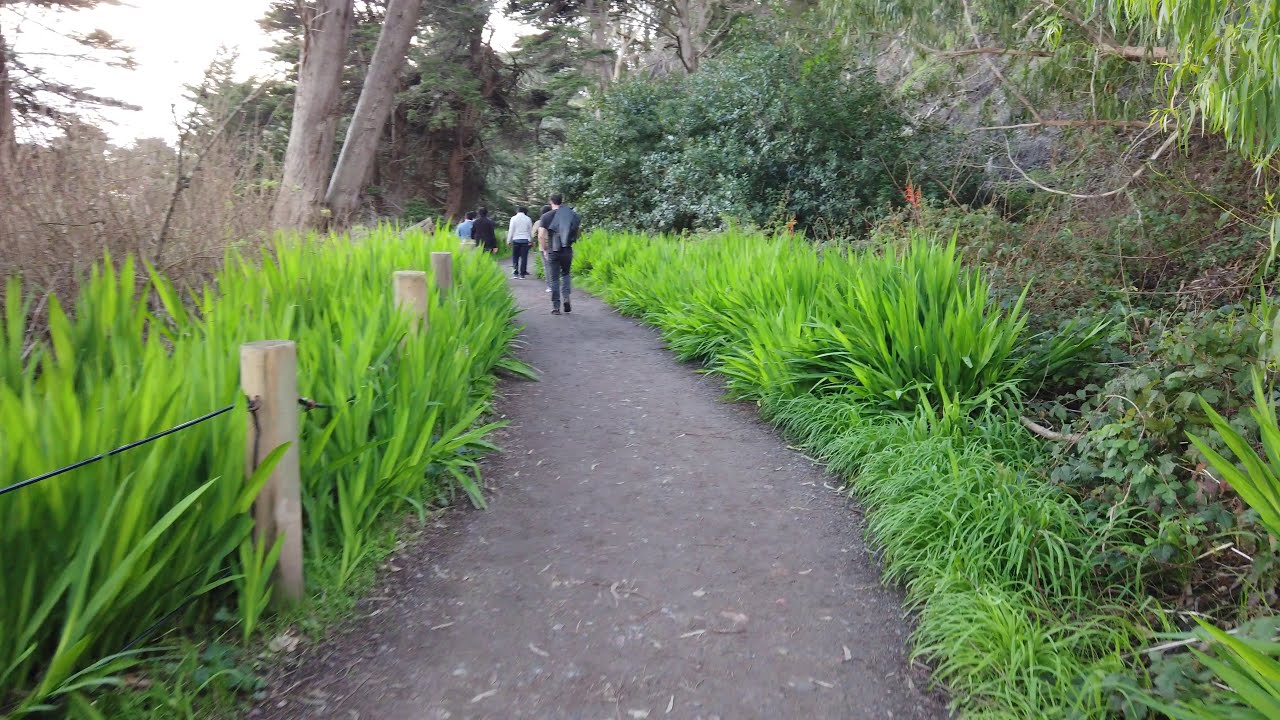This image captures a slightly elevated hiking trail, viewed from a descending perspective. The path, which appears to be a compacted mud walkway, is bordered on both sides by lush, green vegetation that has a jungle-like aspect. On the immediate edges of the trail, there are short bushes and shrubs with long green leaves. To the right, the foliage seems more dense and grows up the side of a hill, adding a slight elevation to that side. Conversely, the vegetation decreases to the left, where a wooden fence composed of vertical posts connected by a single rope or chain runs alongside the trail. Intermixed with the greenery, some downed twigs and dried bushes can be seen, indicating areas of less maintained plant life. Additionally, tall grasses and more trees populate the background, while five people traverse the path, providing a sense of activity and scale to the natural setting.